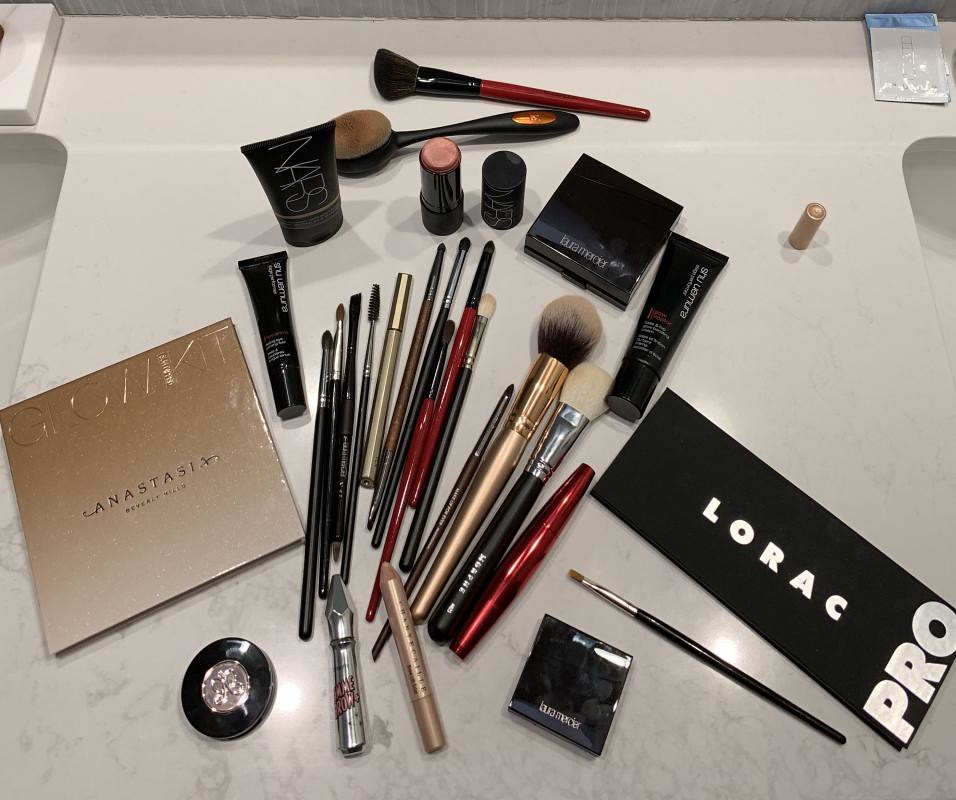This vibrant overhead shot displays an extensive collection of makeup tools and products meticulously arranged. Central in the composition, we see an assortment of eyeshadow brushes of various shapes, each distinguished by unique handles in black, beige, and red. Among these is a mascara wand standing out from the array. Scattered around the brushes are two makeup sponges, or "poofs": one blush brush featuring a black handle with a silver top, and a face powder brush adorned with a gold handle and a matching gold top.

Adding to the ensemble, several eyeshadow palettes make their presence known. Prominently, the Lorac Pro palette sits to one side, its sleek rectangular form marked by the brand name "LORAC" rendered in silver against a black background. On the left side of the brushes lies the Anastasia Glow Kit, likely containing a mixture of bronzing powder and eyeshadow, identified by its soft tan-colored exterior. The overall arrangement provides a comprehensive snapshot of a well-curated makeup collection, reflecting both utility and artistic flair.